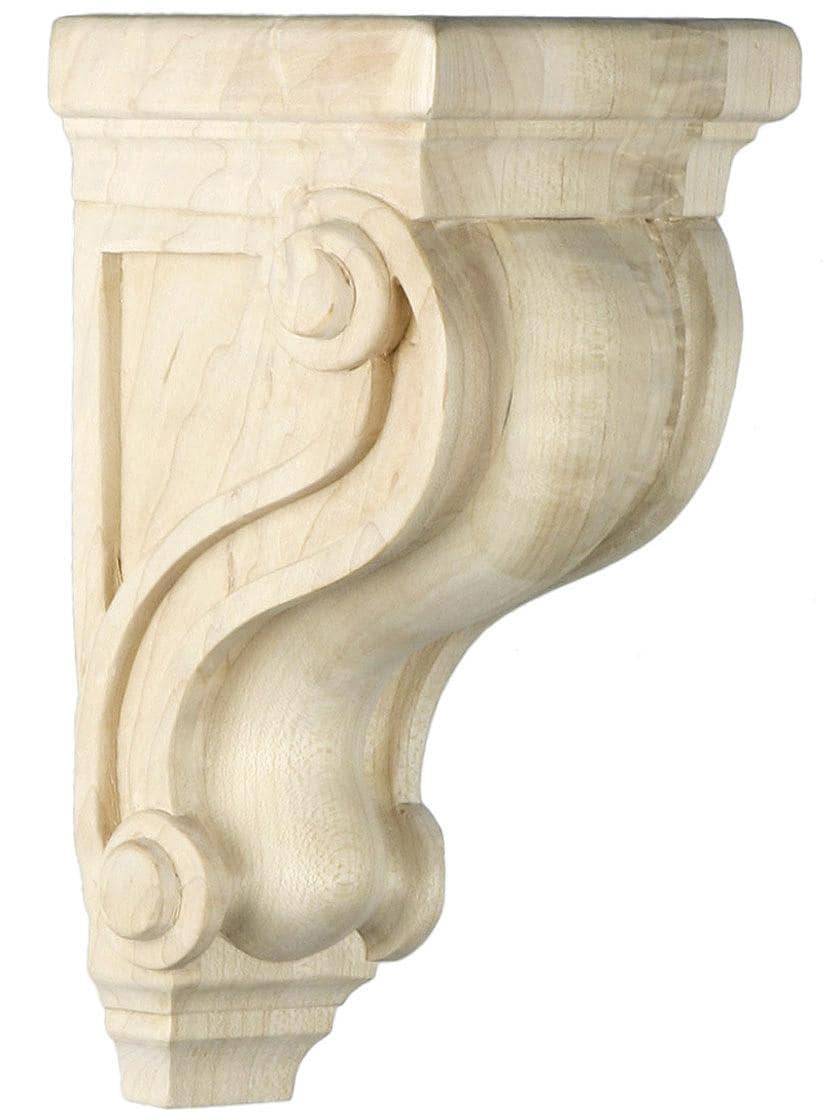The image showcases a meticulously carved object made from light-colored wood, likely birch. The background is a pristine white, emphasizing the natural hue and fine details of the wood. The object features a square base at the top, which transitions smoothly into a curved form that then flares slightly outward. Elegant scrollwork adorns the structure, adding an artistic touch. The visible wood grains suggest it has not been stained, preserving its natural beauty. The surface appears sanded to a fine finish, resulting in a very smooth texture. The left-hand side of the object is perfectly vertical, suggesting it is designed to be mounted on a wall. The flat top surface could serve as a small shelf or support. The construction appears to involve several pieces of this light-colored wood, seamlessly joined together to create a cohesive piece.